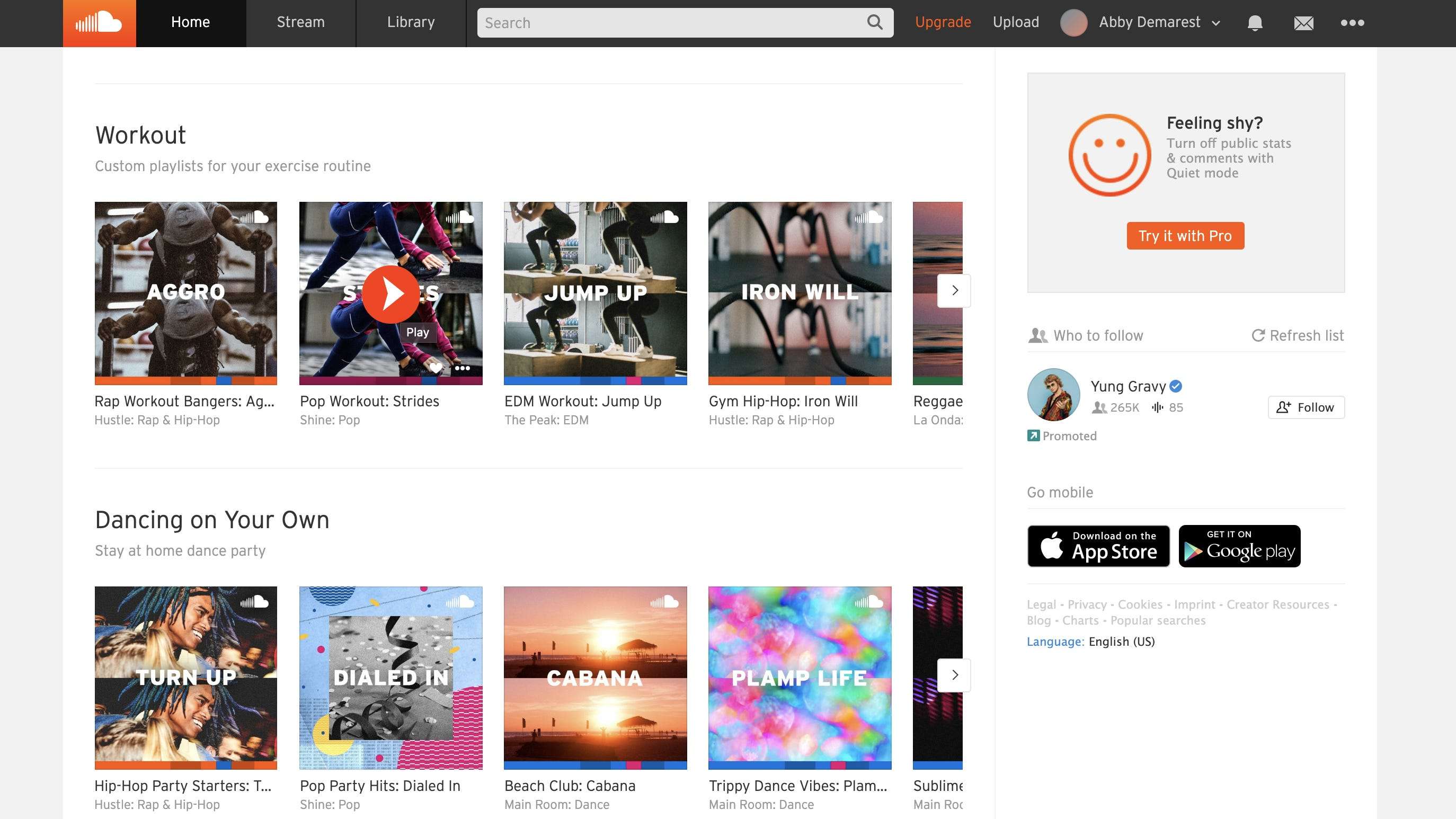This is a detailed caption for the given image of a SoundCloud screenshot:

---

The image is a screenshot of the SoundCloud website, showcasing a variety of songs and playlists available for listening. Dominating the top of the image is a horizontal black bar, which contains the main menu of the website. To the top left of the bar, within an orange box, is SoundCloud’s iconic white cloud logo. Spanning across the top center of the screen, there are multiple options presented, including "Home," "Stream," "Library," a white search box, "Upgrade," "Upload," followed by the account holder's username, and several icons for notifications and settings. The menu options are set against a light gray background, with "Home" highlighted in black to indicate it is the currently selected option. 

The area below the navigation bar features a white background and is divided into sections showcasing different music themes. The first row, titled "Workout," presents four playlist options: "Aggro," "Jump Up," etc. Each option includes an associated cover image. Clicking on any of these options leads to curated playlists designed for workout sessions.

The second row is titled "Dancing on Your Own" and similarly offers four playlist options: "Turn Up," "Cabana," "Plump Life," and "Plamp Life," each accompanied by distinctive, colorful images.

On the right-hand side of the screen, there is a column containing additional information related to the music and the user's account. Featured here is an artist named Young Gravy, who appears to be linked to the current playlist. 

At the bottom of this column are black links directing users to the Apple App Store and Google Play Store, promoting the download of the SoundCloud app for mobile devices.